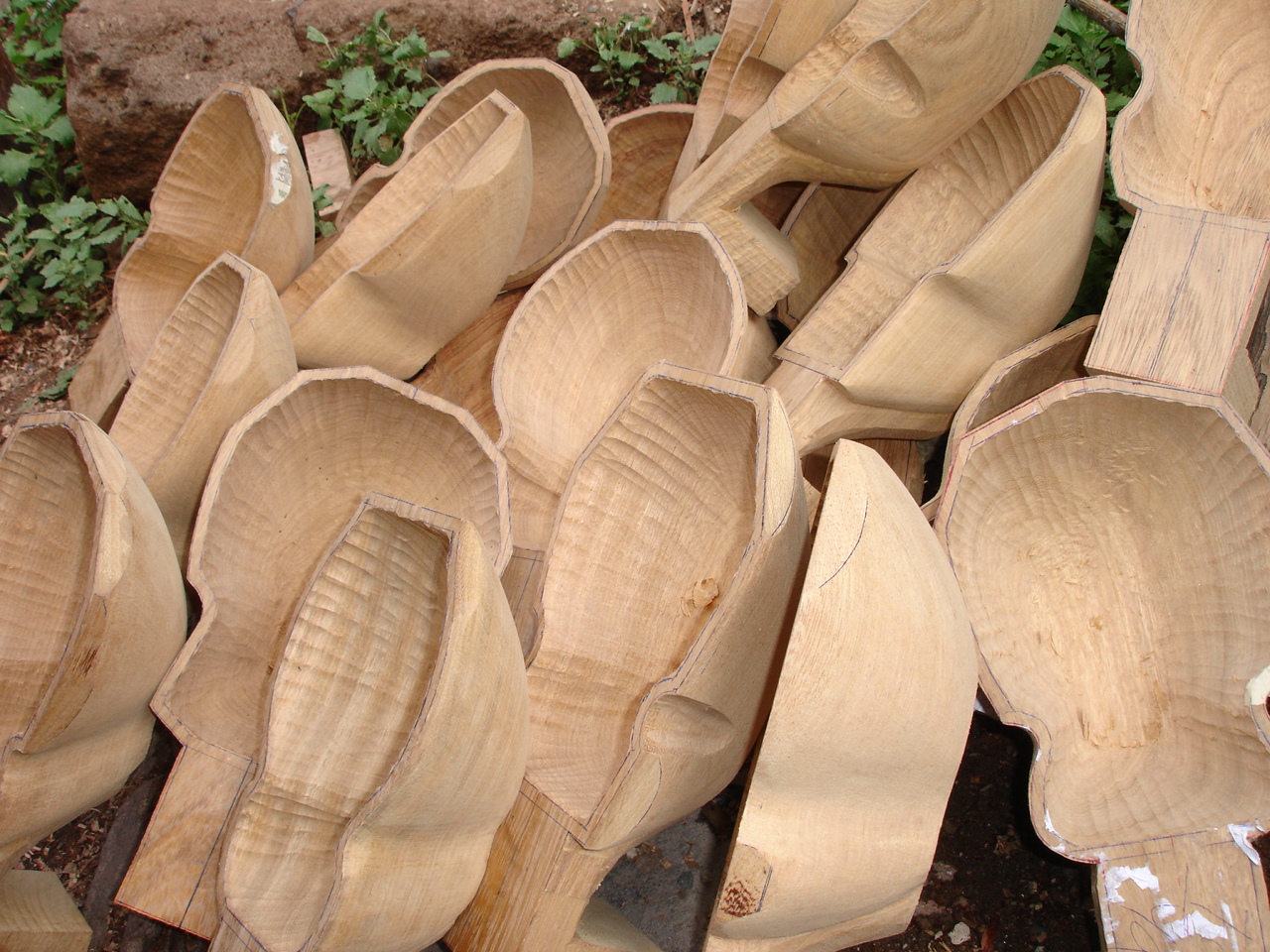In this outdoor image, we see a large, unsystematic pile of small, hand-carved objects that resemble a cross between bowls and scoops, made from unfinished, pale blonde wood. Each piece features a handle and is deeply carved, suggesting a potential use such as creating a small water pond. The intricate carvings inside add texture with random lines. Notably, the one in the lower right corner has some white residue on its handle, with a shiny or lacquered finish atop the grip. The scene is further characterized by its backdrop: in the upper left, there are large, indistinct brown rocks, possibly large boulders or a swath of mud, surrounded by greenery that includes small plants reminiscent of clovers and weeds. The overall arrangement, combined with the natural setting, imparts a somewhat unsettling and disordered feeling.